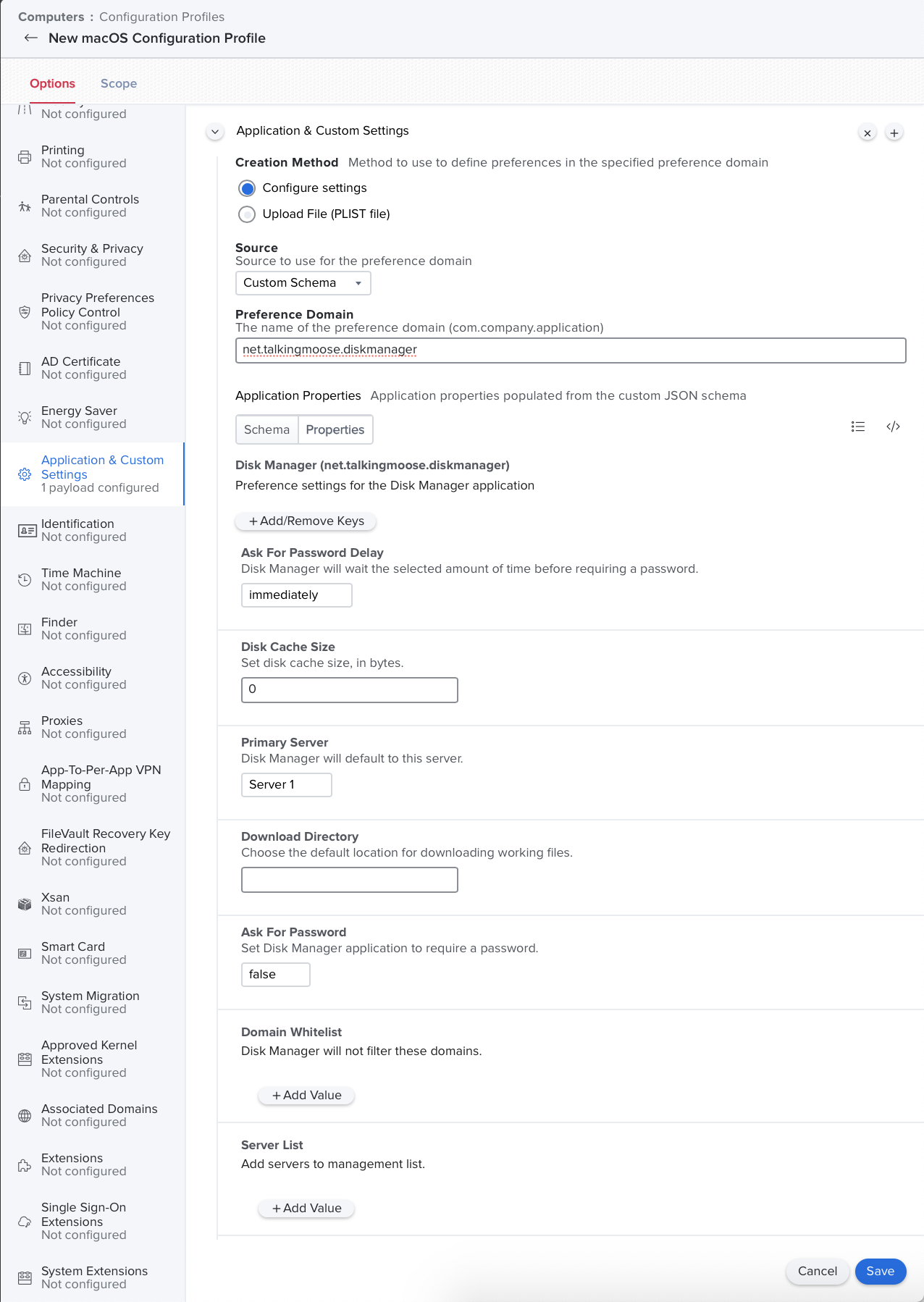The image showcases a lengthy, predominantly light-colored webpage filled with textual content. In the upper left corner, the title "Computers Configuration Profiles" is displayed, with "A New Mac OS Configuration Profile" emphasized in bold text just below it. The webpage features a long left sidebar that includes segmented sections, with the title "Options" underlined in red, and adjacent to it, another section labeled "Scope" in blue.

The main body of the webpage expands on configuration details, listing multiple options accompanied by icons. All options are written in black text, except for "Applications and Custom Settings," which stands out in blue. The content further illustrates a section titled "Application Custom Settings," and guides through the configuration process, highlighting "Configure Settings" under the "Creation Method" in blue.

Additionally, the configuration profile elaborates on several technical elements such as "Source Preference Domain," which is a field filled with an example domain. Other listed components include "Application Properties," "Disk Manager," "Ask for Password Delay," "Disk Cache Size," "Primary Server," "Download Directory," "Ask for Password," "Domain Whitelist," and "Server List." The last two entries, "Domain Whitelist" and "Server List," feature an option to "Add Value" underneath them.